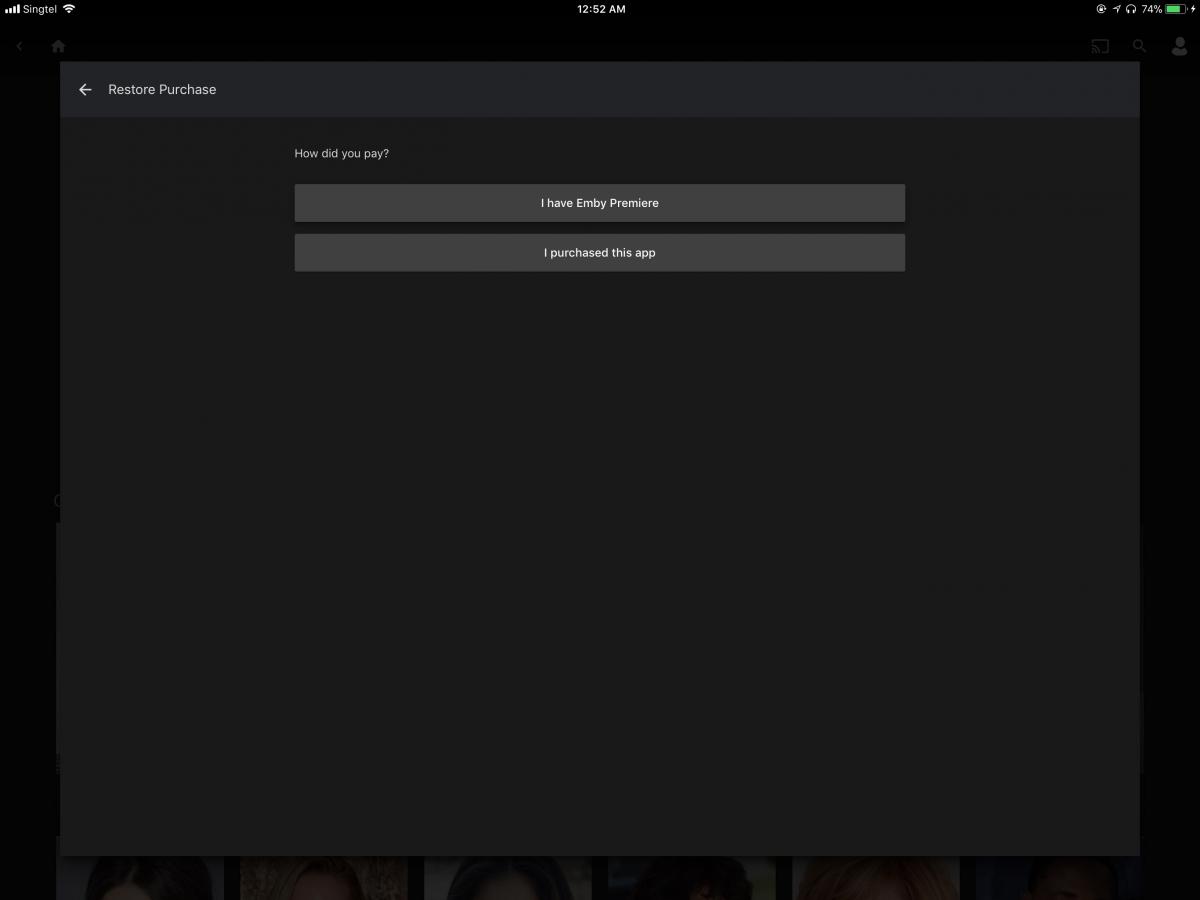The image showcases a dark-mode interface on a device resembling an iPad. The screen prominently features a "Restore Purchase" window with options to select "How did you pay?" Below this, there are two clickable buttons: "I have MB Premiere" and "I have purchased this app." The rest of the page remains predominantly empty, with a "Back" button located near the "Restore Purchase" prompt. The interface likely pertains to retrieving a previously purchased app. The background is dark, and the text appears in white or light gray. The device status bar indicates the current time as 12:52 a.m., with a battery level of 74%, headphones plugged in, and a strong signal. Additionally, there is partially visible text, possibly "5ing NL," in the status bar.